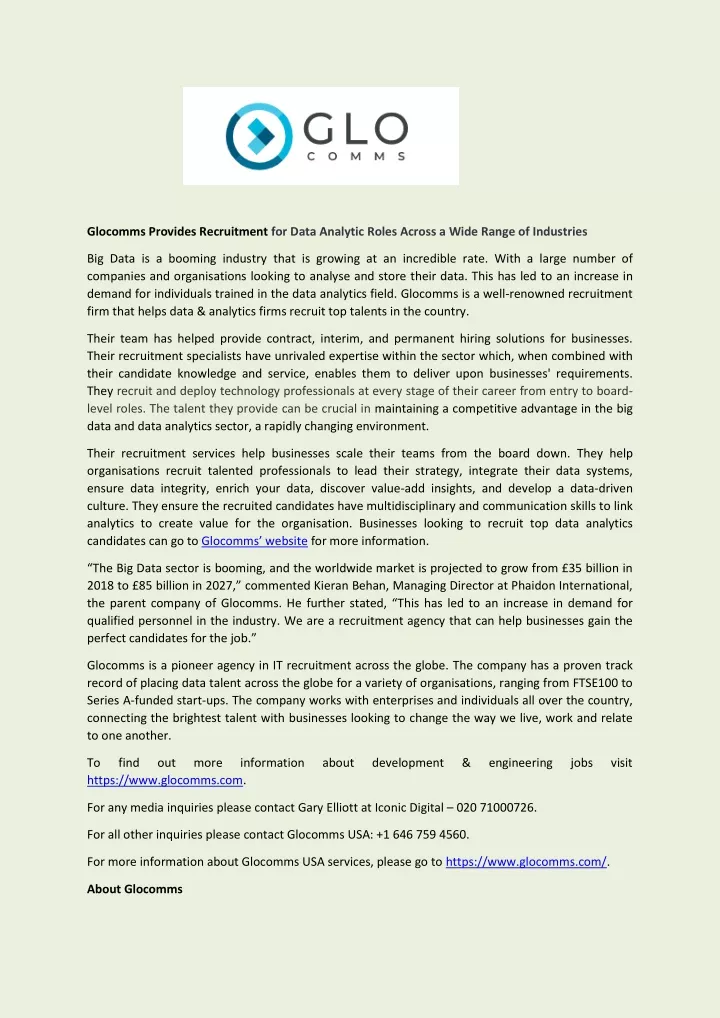**Descriptive Caption:**

On a light green background, this image showcases a letter-style format. At the top, a circular logo in light and dark blue features an arrow pointing to the right, accompanied by the text "Glocomms," spelled out as G-L-O-C-O-M-M-S. The caption highlights that Glocomms specializes in recruiting for data analytics roles across a diverse range of industries.

Glocomms identifies data analytics as a rapidly growing sector, driven by an increasing number of companies seeking to analyze and store their data. This growth has amplified the demand for skilled professionals in data analytics. As a renowned recruitment firm, Glocomms excels in connecting data analytics firms with top talent, offering solutions for contract, interim, and permanent positions. Their team of recruitment specialists boasts unparalleled expertise in the sector, combining deep candidate knowledge and exceptional service to meet business needs.

Glocomms caters to technology professionals at all career stages, from entry-level to board-level roles. The talent they recruit is vital for maintaining a competitive edge in the dynamic big data and data analytics sectors. Their services help businesses expand their teams by recruiting professionals who can lead strategy, integrate data systems, ensure data integrity, enrich datasets, uncover valuable insights, and cultivate a data-driven culture. They ensure candidates possess multidisciplinary skills and effective communication to link analytics with organizational value creation.

Businesses interested in hiring top data analytics candidates can visit Glocomms' website for more details. The big data sector's global market, valued at $35 billion in 2018, is expected to grow to $85 billion by 2027. Kieran B. Hahn, Managing Director of Fabian International, Glocomms' parent company, notes the heightened demand for qualified personnel in the industry. Glocomms prides itself on being a pioneering IT recruitment agency with a proven track record of placing data talent worldwide, from large corporations to agile startups.

For more information about data analytics recruitment, development, and engineering jobs, visit www.glocomms.com. For media inquiries, contact Gary Elliott at Iconic Digital, and for general inquiries, reach Glocomms USA at 646-759-4560. Learn more about Glocomms' U.S. services at www.glocomms.com.